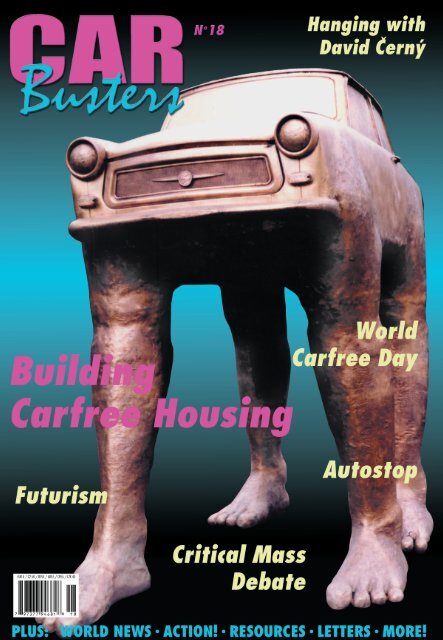The front cover of the magazine titled "Car Busters" prominently displays a striking image of a vintage, rusty car with four sturdy, human-like legs instead of wheels. The car, depicted in shades of brown and grey, appears to be marching, with its feet rendered in a greyish hue. The backdrop features a black gradient at the top and bottom, transitioning to a blue center, creating a dramatic contrast with the central image. Surrounding the car are various text elements in pink, blue, and yellow. The top left corner proudly declares "CAR BUSTERS" with 'CAR' in bold pink and 'BUSTERS' in light blue cursive. The top right corner reads "Hanging with David Cerny," while smaller text at the top center indicates "n18." Scattered throughout the cover are phrases such as "Building Car-Free Housing," "World Car-Free Day," "Autoshop," "Futurism," and "Critical Mass Debate." At the bottom, a light blue text reads, "Plus World News, Action, Resources, Ledgers, More." A barcode is positioned in the bottom left corner, adding an element of typical magazine formality to this eye-catching and thought-provoking cover.